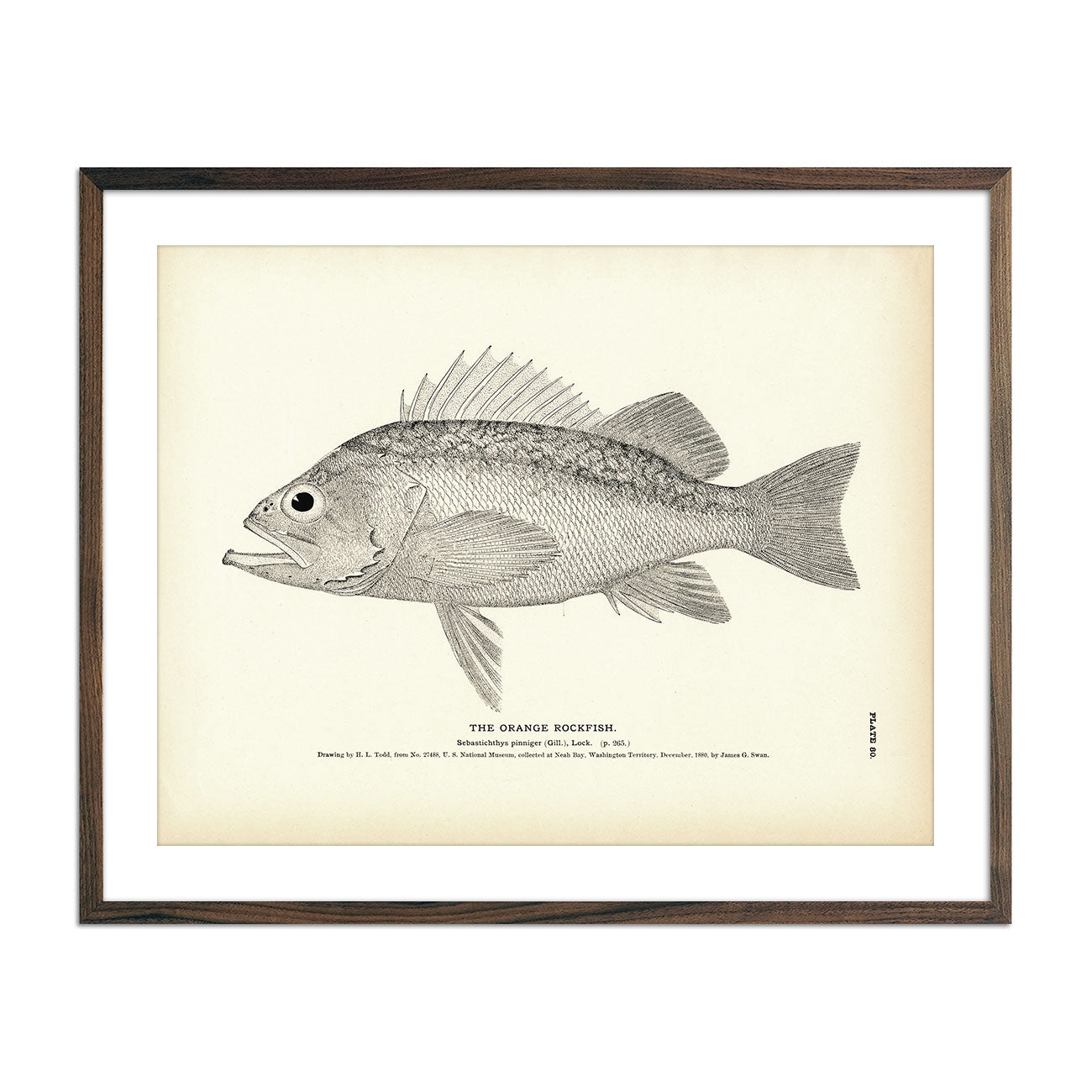The image depicts a detailed, black-and-white illustration of an "orange rockfish," reminiscent of those found in old biology textbooks. This side view illustration is placed on a yellow-aged page, bordered by a white mat within a thin wooden frame. The fish, with its left side exposed, features a distinctive set of spiny dorsal fins on top, followed by a seashell-shaped fin near its tail fin. There are multiple fins, including a prominent one on the center-bottom and arm-like fins extending from the sides. Its scales transition from very small to larger ones towards the top back portion. The illustration includes intricate details like the jagged gill, large open mouth with a protruding lower jaw, and a black eye. Below the fish, in black text, is the label "the orange rockfish," followed by more fine print that is partially legible, mentioning details such as "Sebastophe's plinger," "Gillilock, Washington Territory," and a date difficult to discern.